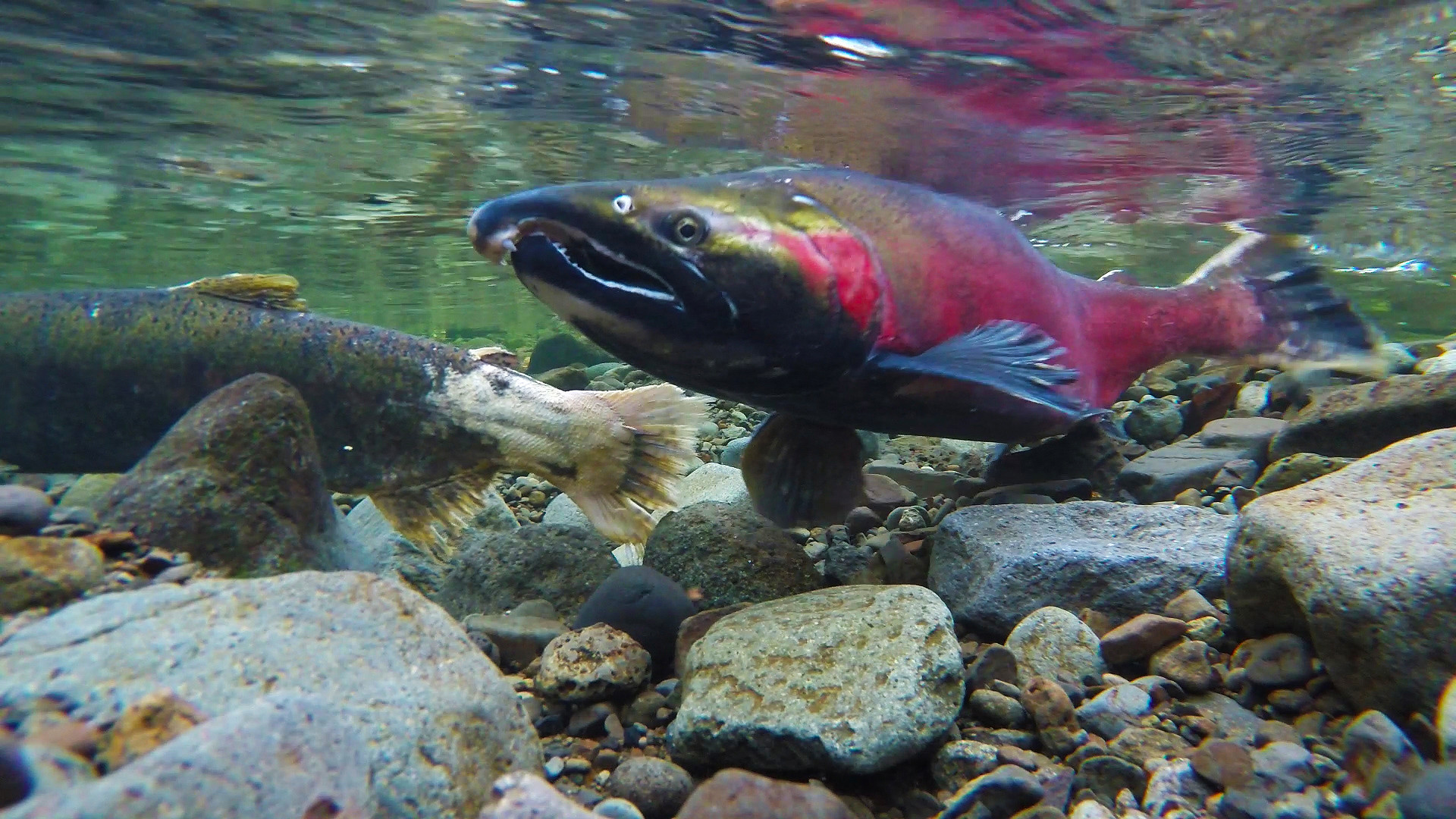This photograph captures two distinctly colorful fish swimming in a shallow, clear stream, teeming with a variety of rocks and pebbles. The water is so shallow that the dorsal fin of the fish in the foreground appears to be breaking the surface. This fish, with a distinctive hooked snout and sharp teeth, flaunts a striking cranberry-red body with a green head, black front fins, and a stark black tail. This vivid creature resembles a salmon, particularly notable for its post-spawning chum phase, where its vibrant colors contrast with the fading white patches. The second fish, only partially visible with its greenish-brown body and white tail, appears a different species. The streambed is a visually rich mosaic of large rocks, smaller stones, and patches of mud, all rendered in sharp detail by the crystal-clear water, which provides an unobstructed view all the way to the bottom, suggesting a depth of six to eight inches. The photograph, much wider than it is tall, evokes a sense of tranquility in this rustic underwater scene.